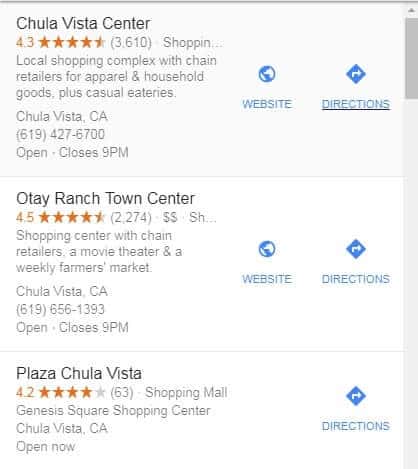A pixelated and low-resolution image, likely from a Google Maps search, displays three shopping centers in Chula Vista, California, each accompanied by details such as ratings, reviews, and operational information.

1. **Chula Vista Center**: Rated at 4.3 stars based on 3,610 reviews, this establishment is currently open and will close at 9 p.m. The listing includes a phone number and provides links to both its website and directions.

2. **Otay Ranch Town Center**: With a rating of 4.5 stars from 2,274 reviews, this slightly more upscale option (indicated by two dollar signs) is also situated in Chula Vista. It is currently open and also closes at 9 p.m. The description includes a phone number as well as links to the center's website and directions.

3. **Plaza Chula Vista**: This location holds a 4.2-star rating from 63 reviews. It is currently open and provides a link for directions. The description mentions that it is located in Chula Vista, California.

All three listings offer additional text with descriptions and operational statuses, helping users decide on their shopping destination.